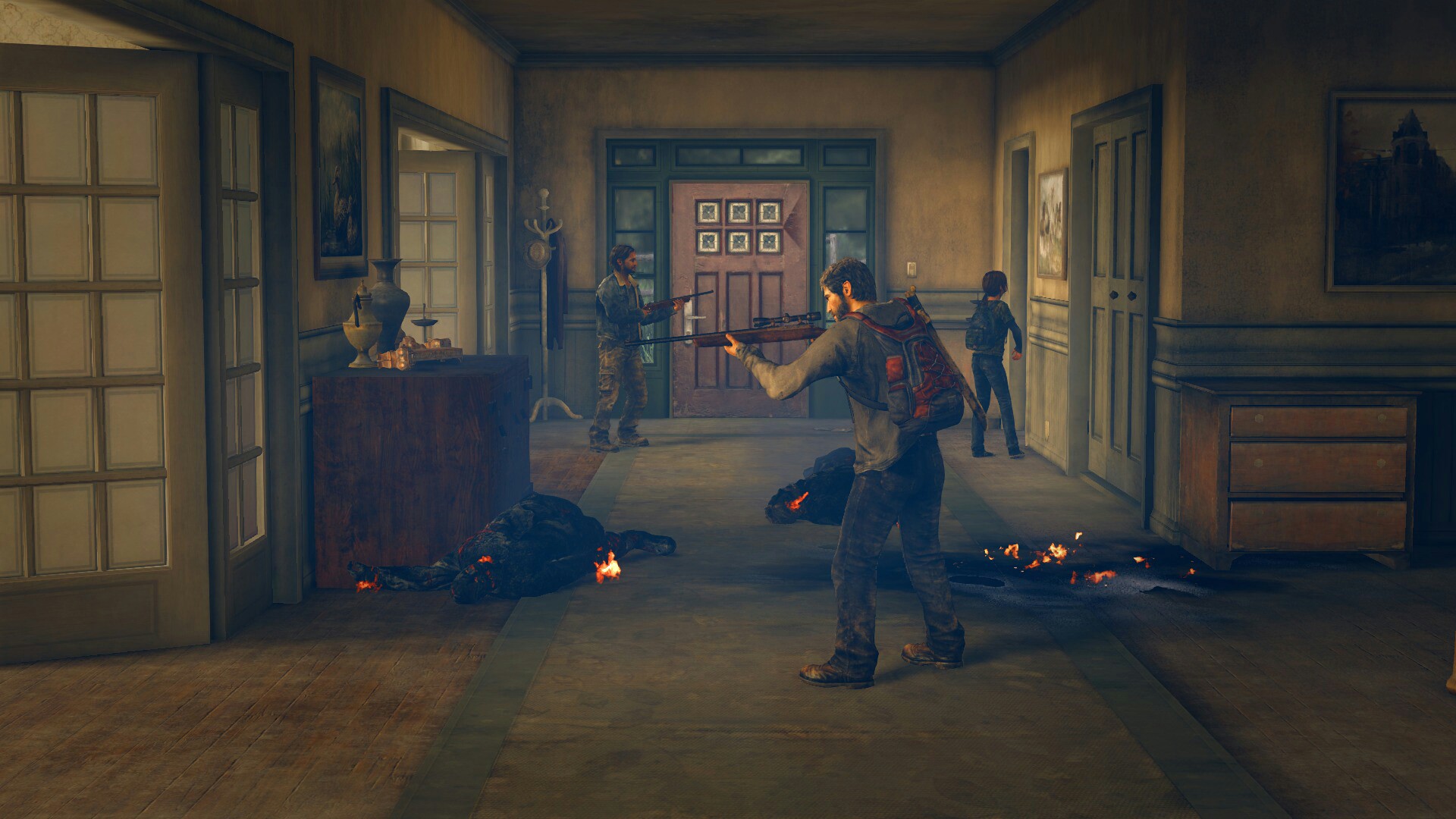A tense scene unfolds within a dimly lit, expansive corridor interior bathed in a dingy khaki hue. Three men are visible within the frame, the nearest of whom carries a rucksack on his back. The middle figure, along with the man further down the corridor, are both aiming guns forward, creating an atmosphere laden with danger. Strewn across the floor are mysterious objects that might be lifeless bodies, adding to the chilling tension of the setting. On the right side of the image, flames can be seen flickering ominously, casting a dire glow on their surroundings. A person in the distance walks towards what appears to be a solid wall, though it might conceal a doorway, suggesting a sense of urgency or escape. The left side of the corridor features a sideboard with a vase, hinting at a once normalcy now overshadowed by the prevailing chaos. The lack of light further accentuates the grim mood pervading the space.